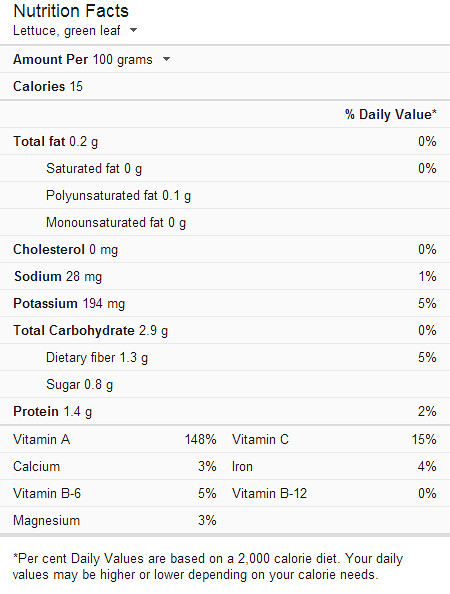This image displays the nutrition facts for green leaf lettuce, presented in a clean and precise format, likely sourced from an online screenshot rather than a physical photo. The nutritional information is based on a 100-gram serving size, detailing the following:

- **Calories**: 15 kcal
- **Total Fat**: 0.2 grams
  - **Saturated Fat**: 0.0 grams
  - **Polyunsaturated Fat**: 0.1 grams
  - **Monounsaturated Fat**: 0.0 grams
- **Cholesterol**: 0.0 milligrams
- **Sodium**: 28 milligrams (1% DV)
- **Potassium**: 194 milligrams (5% DV)
- **Total Carbohydrates**: 2.9 grams
  - **Dietary Fiber**: 1.3 grams (5% DV)
  - **Sugars**: 0.0 grams
- **Protein**: 1.4 grams (2% DV)

In terms of vitamins and minerals, green leaf lettuce offers substantial nutrients:
- **Vitamin A**: 148% DV
- **Calcium**: 3% DV
- **Vitamin B6**: 5% DV
- **Magnesium**: 3% DV
- **Vitamin C**: 15% DV
- **Iron**: 4% DV
- **Vitamin B12**: 0% DV

These percentage daily values (DV) are based on a 2,000-calorie diet, and individual nutritional needs may vary.